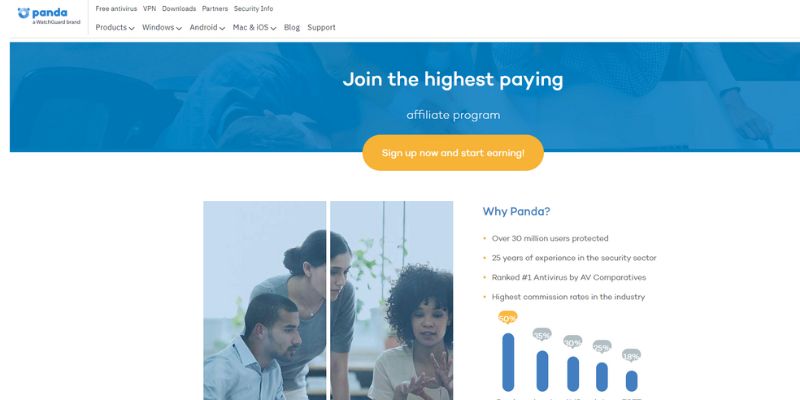This image depicts the homepage of a website for Panda Security, a company specializing in antivirus and malware protection for various devices. At the upper left corner, a blue logo featuring a stylized panda is displayed, with "WatchGuard" written underneath in black text. The top navigation bar offers categories such as Free Antivirus, VPN, Downloads, Partners, Security Info, and a Products drop-down menu indicating options for Windows, Android, Mac, and iOS platforms. Additional sections include a Blog and Support.

Central to the page is a prominent blue rectangular banner promoting an Affiliate Program. The banner reads, "Join the highest paying affiliate program," complemented by a yellow "Sign Up Now and Start Earning" button. The background features a generic office setting, creating a professional and inviting atmosphere.

Below this, another image shows three individuals in an office environment. They are medium-skinned with black hair: a man in a blue shirt, a woman with her hair pulled up wearing a grey shirt, and another woman with curly hair gesticulating as she talks. 

The section titled "Why Panda?" highlights key selling points of the service: over 30 million users protected, 25 years of experience in the security sector, recognition as the number one antivirus by AV Comparatives, and the highest commission ratios in the industry. A bar graph at the bottom of this section shows Panda's commission rate at 50%, significantly higher than the competitors’ figures of 35%, 30%, 25%, and 18%.